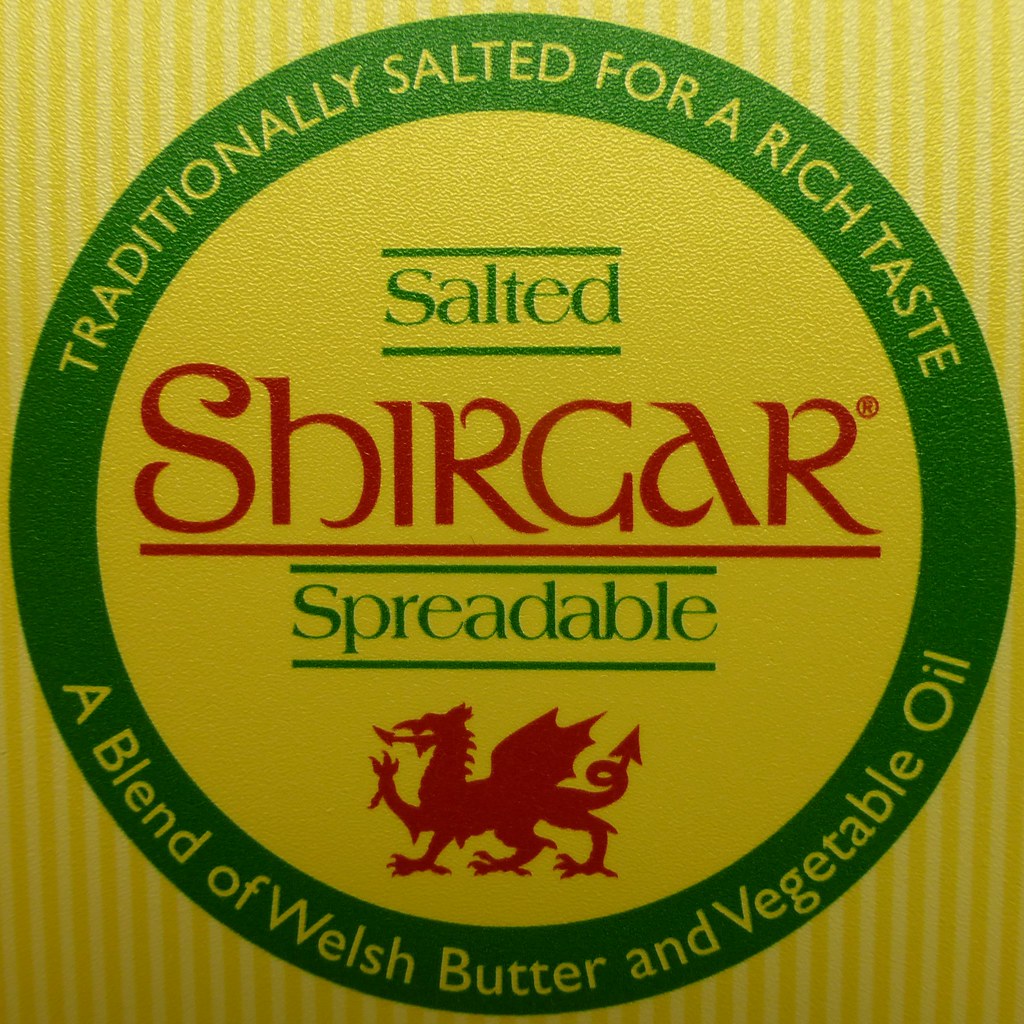The photograph depicts a detailed close-up of a product packaging. The background features yellow and white vertical stripes. Centrally, there is a prominent green circular logo with a yellow inner circle. The green outer circle contains the text "Traditionally salted for a rich taste, a blend of Welsh butter and vegetable oil" written in a circular pattern in yellow. Inside the yellow circle, the word "Shirgar" is displayed prominently in large, old-school red letters. Above "Shirgar," the word "salted" is written in green, and below it, the word "spreadable" is also in green. Beneath this text, there is an image of a red dragon, complete with fire-breathing and an arrow-shaped tail, representing the company logo.